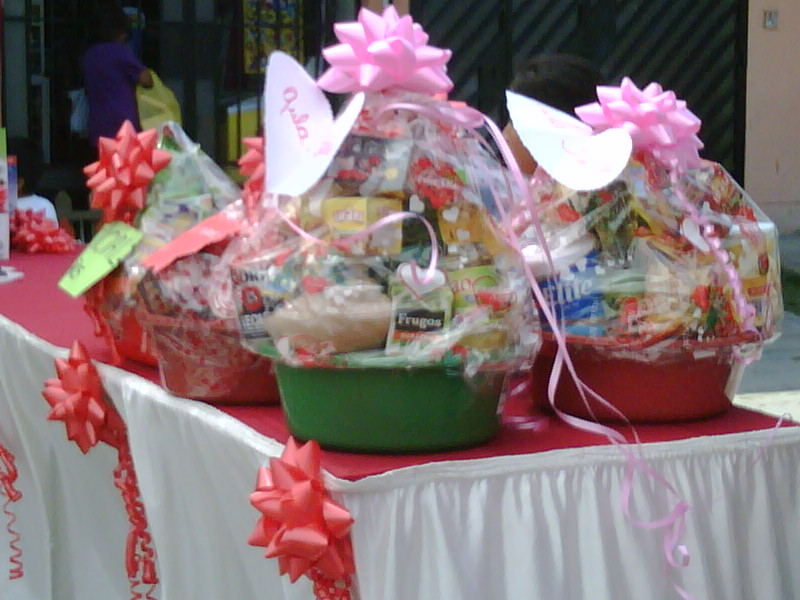This image features a table adorned with a white satin tablecloth that cascades gracefully over the sides, topped with an overlaying red plastic cover. The table is festooned with large red gift ribbons, resembling those used for birthday or Christmas presents, with curly ribbons dangling from them. Several baskets, reminiscent of raffle or prize baskets, are arranged on the table. These baskets, which are filled with a variety of items including products labeled with "Frugos" and "Elite," are wrapped in cellophane and topped with bows in varying colors of red and pink. The baskets themselves are also colorful, with three being red and one green. Each basket has a piece of paper attached to it. In the background, a person wearing a purple shirt and holding something yellow is visible, indicating that this scene is set outdoors next to a doorway.